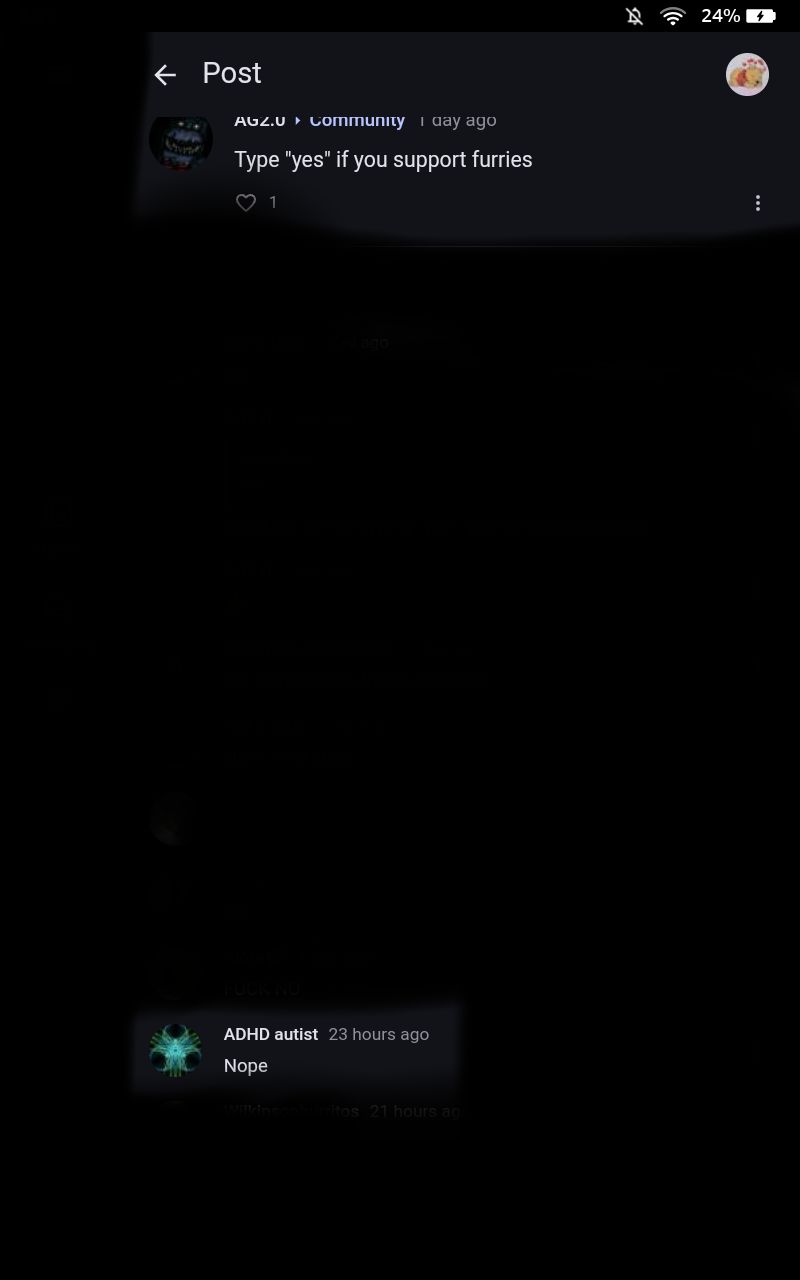In this image, a cell phone screen is displayed against a black background. At the top left corner, white writing shows an alarm icon indicating it is turned off. Next to the alarm, a Wi-Fi signal is almost full, and a battery meter reads 24%. In the middle at the top, a box with an arrow pointing to the left is labeled "Post."

Below this, there is what looks like a Reddit post. It features an image along with a username and community name. To the right of these details, it states the post was made "1 day ago." The main content of the post reads, "Type yes if you support furries," accompanied by another small thumbnail icon in the right corner.

At the very bottom of the image, a comment is visible. It shows an icon associated with the user "ADHD Autist" who commented "23 hours ago," simply saying, "Nope."